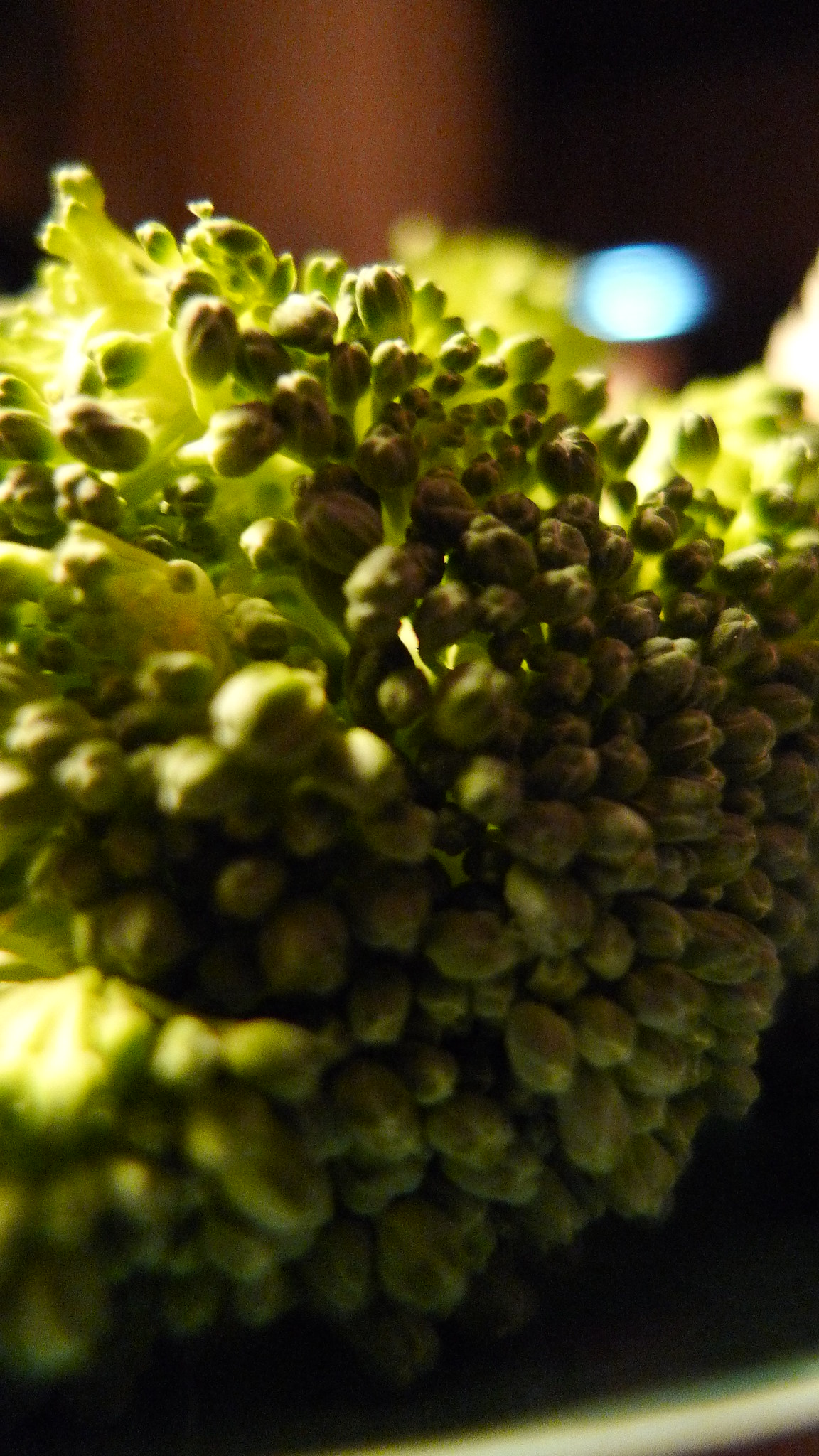This image captures a detailed close-up of a peculiar green plant that takes up about four-fifths of the frame. The plant, reminiscent of a broccoli head when closely examined, features clusters of small green buds of varying sizes sprouting from its stems. The scene is sharply focused on the mid-right section of the plant, accentuating the intricate texture and color of the buds. The background is heavily blurred, revealing only faint outlines of a brown wooden surface or wall and hints of blue light. The plant sits on an indistinct surface with a white border, though the bottom half of the image is entirely black, possibly cast in shadow by the plant under backlighting. The overall appearance suggests a natural, somewhat mysterious botanical subject highlighted against a contrasting backdrop.